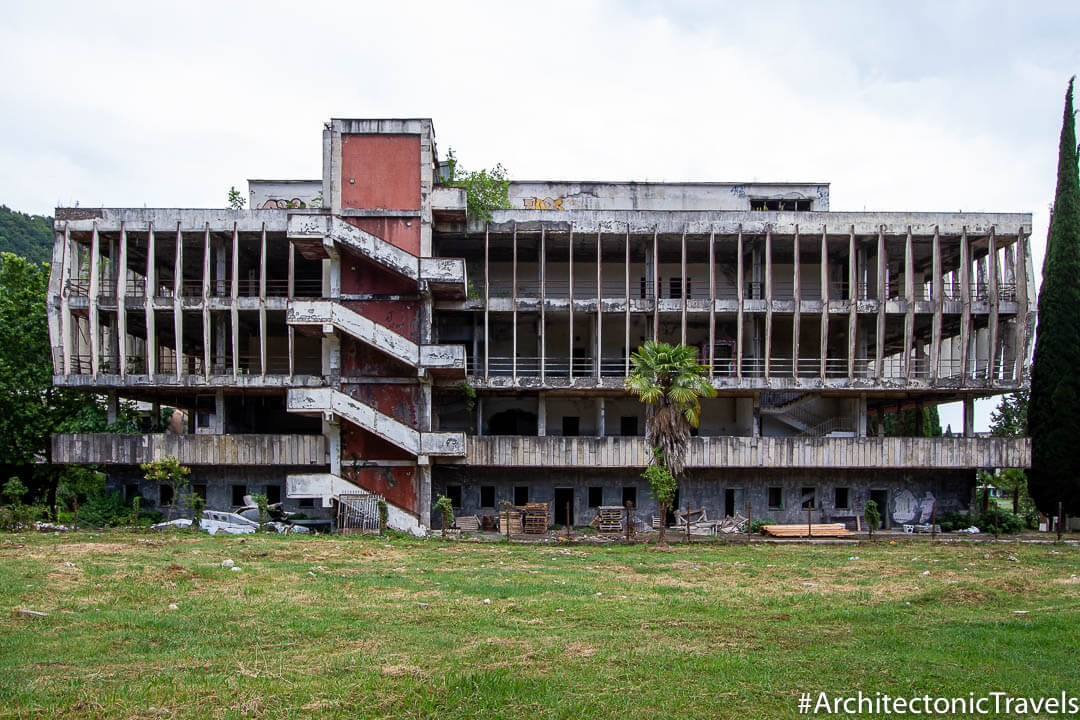The image depicts a severely dilapidated multi-story building, at least five levels high, with pronounced structural decay. The building lacks walls or windows on the side facing us and features distinct vertical pillars between two floors. Prominently, a large ramp fire escape spirals around a central tower, climbing from ground level up to the top. A smaller, decrepit penthouse sits atop the building, and the entire structure is overwhelmed by vegetation, including bushes growing on the roof and base, as well as small trees sprouting from various levels. The middle-left section shows four stairways ascending from the right-hand side. In the foreground, a small fan palm tree reaches up to the third floor, with grass at the building's base. Graffiti decorates the upper portion, and the backdrop is mainly cloudy. The image includes the caption “#architectonic travels” in white text at the bottom.